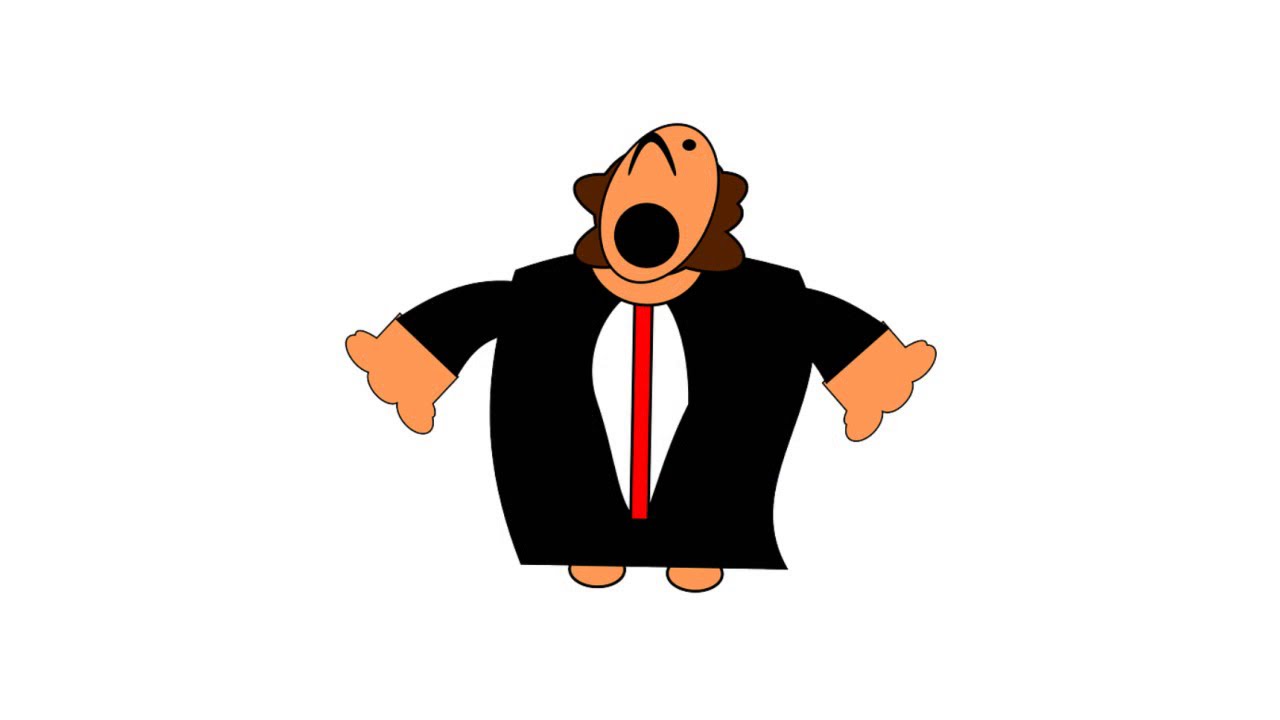The image is a low-quality cartoon clipart of a character that closely resembles a priest or a pastor. It depicts a man with an oval-shaped, peachy tan head, tilted back with his nose—a boomerang-like shape—upturned. His mouth is a wide open black circle, giving the impression that he might be singing, perhaps in a choir or an opera. One black circle eye is visible, while the other is obscured by his large nose. The character has brown hair that bubbles out from the sides of his head.

He wears a long, black coat that extends down to his feet, with long sleeves. The coat is slightly opened in the middle, revealing a white shirt beneath with a thin red tie. His hands are simplistic, depicted as blocky shapes with three large fingers each, and his feet are represented by two round ovals at the bottom. The background of the image is completely white, emphasizing the character's simplistic and cartoonish features. The overall attire is quite square and cylinder-like, providing a somewhat boxy appearance to the entire figure.